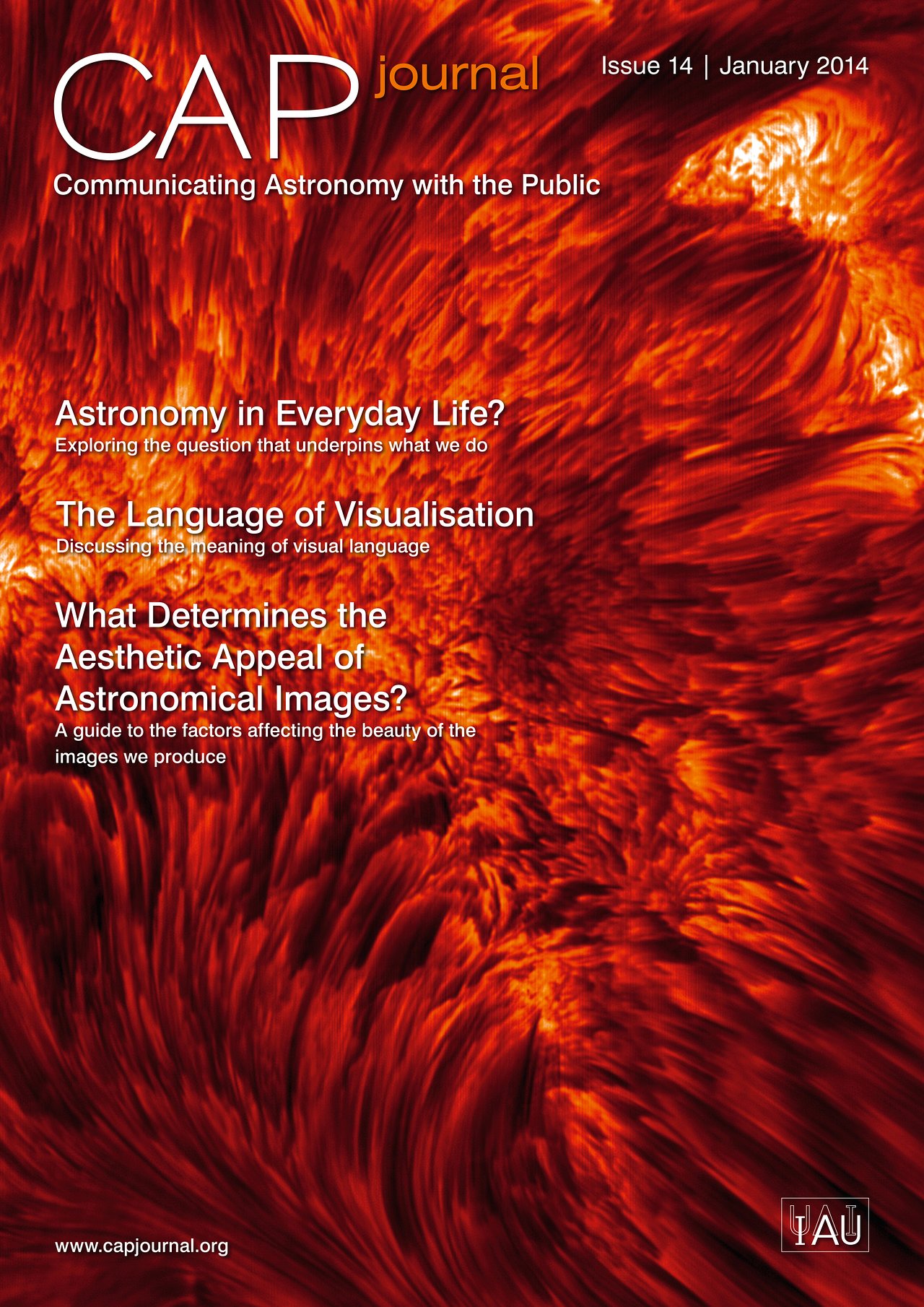This is the cover of the CAP Journal, issue 14, dated January 2014, themed around Communicating Astronomy with the Public. The background features striking red waves that resemble flowing lava or the dynamic flows seen on the surface of the sun. Large, bold capital letters spell out "CAP" on the left, with "Journal" in orange next to it. The cover includes various thought-provoking article titles such as "Astronomy in Everyday Life: Exploring the Question that Underpins What We Do," "The Language of Visualization: Discussing the Means of Visual Language," and "What Determines the Aesthetic Appeal of Astronomical Images: A Guide to the Factors Affecting the Beauty of Images We Produce." At the bottom left, the website www.capjournal.org is listed, and an icon at the bottom right displays the letters IAU, indicating the International Astronomical Union.